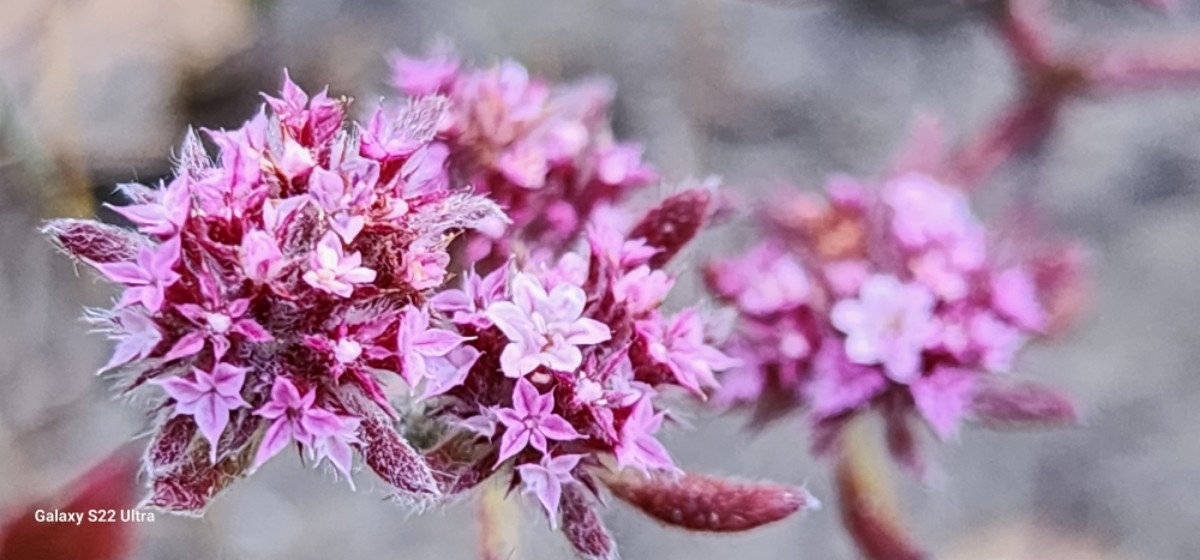This image is a detailed and vibrant photograph showcasing the photography capabilities of the Galaxy S22 Ultra, indicated by the text in the lower left corner. The primary elements in focus are an array of small, delicate flowers predominantly in shades of pink and white. The pink flowers vary in depth, with some displaying dark pink hues while others are lighter. The petals are notably tiny, contributing to the intricate texture of the scene. The leaves of the plants are purplish, almost reddish, adding a rich contrast to the color palette. The background is intentionally blurred, rendering it a soft gray that highlights the sharpness and vividness of the flowers in the foreground. This selective focus technique emphasizes one particular flower as the main focal point, with others slightly out of focus, enhancing the depth of field. Overall, the photograph exemplifies modern photographic techniques by highlighting the toughness of the plant's stem juxtaposed with the tenderness of the flowers, creating a striking visual composition.